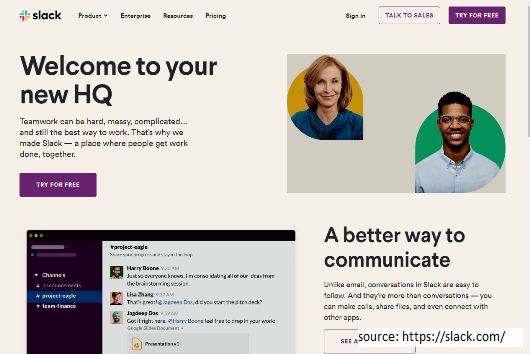The image depicts the Slack homepage, showcasing a user-friendly interface designed to attract potential users. The top navigation bar features several options: a product drop-down menu, enterprise resources, pricing details, and a sign-in button situated on the far right. The sign-in button is black, whereas the "Talk to Sales" button is prominently displayed in purple with a faint purple border. Another key call-to-action, "Try for Free," is also highlighted in purple.

Dominating the left side of the image in large, bold font is the phrase "Welcome to your new HQ." Below this, in smaller text, it reads: "Teamwork can be hard, messy, complicated, and so the best way to work. And that’s why we made Slack, a place where people get work done together." Beneath this message, another "Try for Free" button in purple encourages immediate engagement.

The right portion of the image features two individuals: a Black man positioned at the bottom right with a green circle backdrop. He wears glasses and a light denim dress shirt. In the top left corner is a mid-50s smiling woman with medium red hair wearing a turquoise shirt.

A text block underneath these images states, in larger font, "A better way to communicate." Further elaborated in smaller text, it reads: "Unlike email, conversations in Slack are easy to follow, and there are more conversations. You can make calls, share files, and even connect with others."

The bottom of the image appears to have additional text obscured by a watermark reading "source slack.com." To the left, another section contains a screenshot displaying a Slack channel interface on an Apple device, likely a Mac. This screenshot includes three dots at the top and various tabs on the left side, along with snippets featuring three different individuals and brief descriptions presumably explaining their roles.